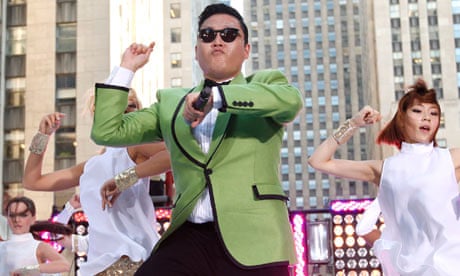The image is a vibrant color photograph of an Asian man, possibly Korean, performing a dance routine on stage, reminiscent of the Gangnam Style dance from South Korea. He stands confidently in the center, wearing a green blazer, white shirt, black trousers, and dark sunglasses. His right arm is raised at a 90-degree angle upwards, with his hand near his head, fingers closed, while his left hand holds a microphone pointed towards his chest. His black hair is neatly styled, and his mouth is closed, focusing on the performance.

Behind him, two backup dancers, also Asian women, are positioned. The dancer to his left is dressed in a white sleeveless outfit, and the dancer to his right is in a similar white dress, adorned with red hair and hands raised to the side of her head. They perform energetically in sync with him. The backdrop features a tall office building with distinct lights at the bottom, emitting purple and white hues, adding a dynamic urban feel to the scene, as if they are performing for a major TV show in a bustling downtown city setting.